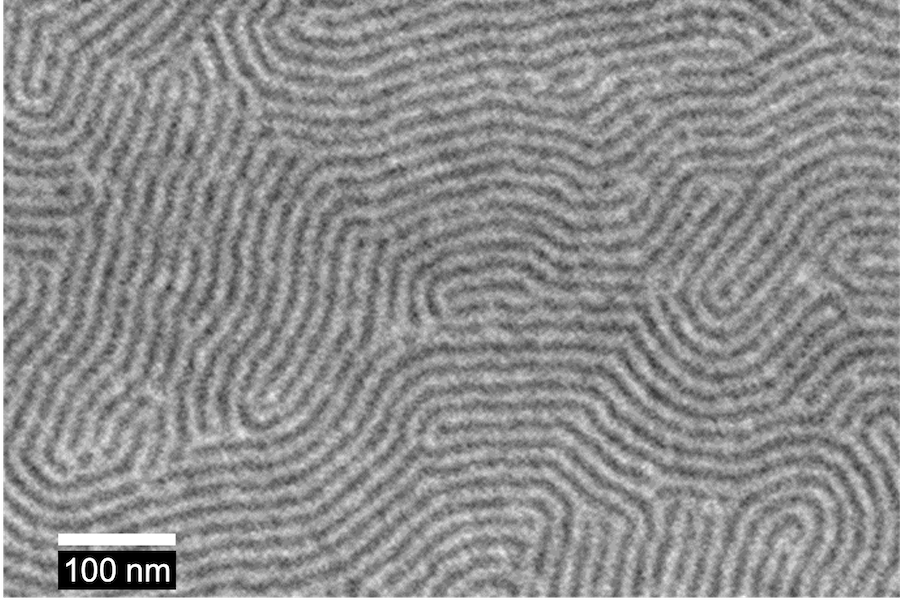The image is an extremely zoomed-in, microscopic photograph showcasing a highly magnified structure that resembles random, overlapping swirls of gray-colored lines with black borders, reminiscent of carbon nanotubes or a fingerprint but without a central point of reference. The predominant colors are white, gray, and black, rendering the structure in a blurry and pixelated manner against a white background. The rectangular photograph features a small scale indicator in the bottom left corner, consisting of a thinner white rectangle above a black rectangle. The black rectangle contains white text that reads "100NM," denoting a measurement of 100 nanometers.